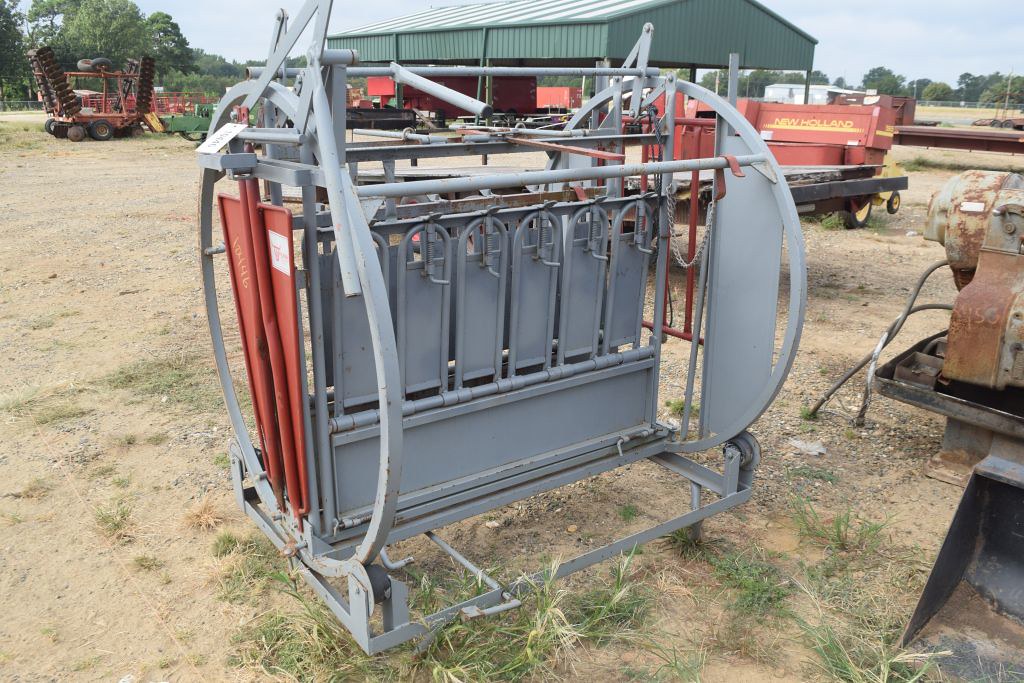In this color photograph, the focal point is a large squarish grey metal object identified as a livestock table, centrally framed with additional metal structures. The table, which appears complex with cylindrical outlines and a metal frame encompassing it, is used for handling animals during veterinary procedures or transportation. Flanking the table are red metal beams, one of which contains a white label. The parched, beige ground beneath it features sparse patches of green grass and areas of grey gravel. To the right, a rusted piece of machinery with dangling wires is visible. In the background, the roof of a green barn shelters various pieces of farming equipment, and there’s a red truck or trailer with yellow, illegible writing nearby. The upper left corner reveals another piece of farm machinery, possibly a tractor. The scene is completed with distant trees and a partly visible blue sky, contributing to the image of a hardworking, rural farm setting.